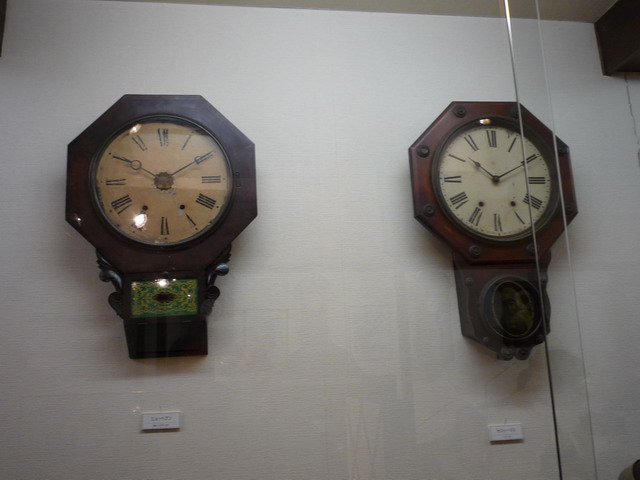The image showcases two hexagonal clocks mounted side by side on a white wall, both encased behind clear glass. At the bottom of the glass panel, a faint reflection of a person is visible. The clocks share a dark wooden finish, but exhibit distinct differences in design. 

The clock on the right is primarily yellowish-brown with Roman numerals embedded in a circular formation within the hexagon. It has small decorative circles adorning each corner of the hexagon. Below this clock there's a small rectangle featuring a green and yellow pattern, which is framed by wooden detailing. A brown rectangular base, possibly part of the clock's stand, is situated underneath this patterned rectangle.

In contrast, the clock on the left is white and lacks the corner circles present on the other clock. This clock has a distinctive piece at the top resembling a square with an attached circle, leading into the clock face that also displays Roman numerals. The middle of the clock face features two hands pointing to indicate the time.

Both clocks rest above a small white plate with illegible writing, adding a touch of mystery and elegance to the overall arrangement.